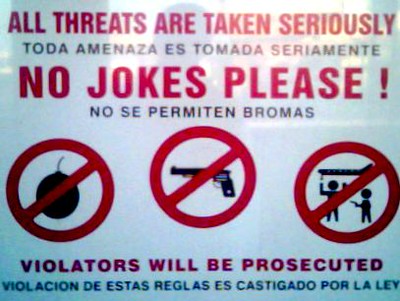The image is a photograph of a warning sign posted against a reflective white surface, and possibly behind glass, resulting in a slightly blurred and pixelated appearance. At the top of the sign, in large red capitalized letters, it reads "ALL THREATS ARE TAKEN SERIOUSLY." Directly below this, in black text, is the Spanish translation, "TODA AMENAZA ES TOMADA SERIAMENTE." Following this, also in red letters, it states, "NO JOKES, PLEASE," with its Spanish equivalent, "NO SE PERMITEN BROMAS," underneath. 

The middle section of the sign contains three red circles, each with a diagonal red line through them, indicating prohibition. From left to right, the symbols inside the circles depict a bomb, a gun, and a person pointing a gun at another individual with an airplane overhead. At the bottom of the sign, in red text, it warns "VIOLATORS WILL BE PROSECUTED," followed by the Spanish translation, "VIOLACIÓN DE ESTAS REGLAS ES CASTIGADA POR LA LEY." The reflective surface of the sign renders some faint, shadowy human shapes, adding to the overall depiction of the photograph.